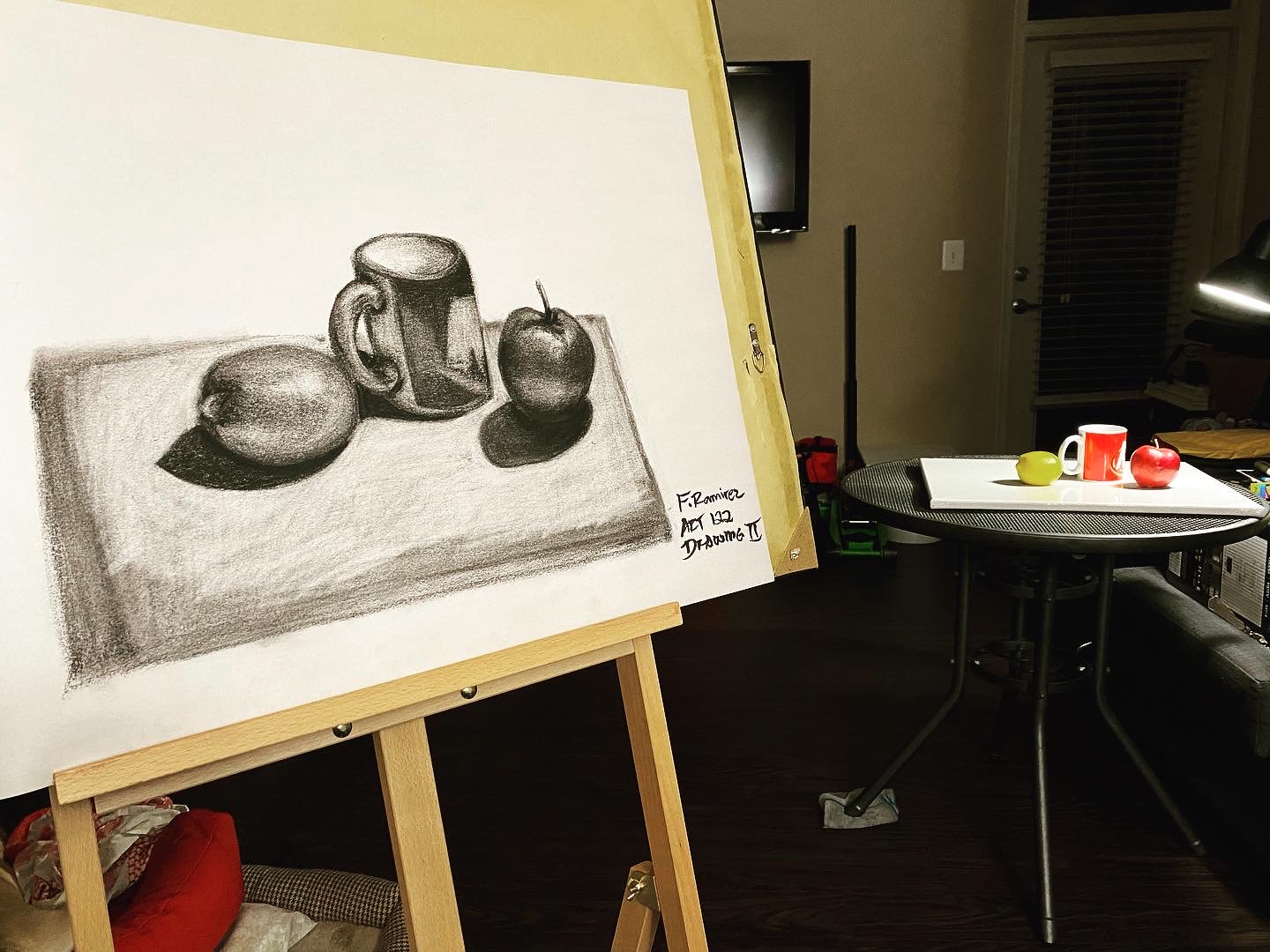Indoor color photograph. The image prominently features a light brown wooden artist's easel positioned towards the left, partially cut off by the left edge and angled into the background. Resting on the easel is a large rectangular piece of white paper displaying a detailed black-and-white pencil sketch. The sketch depicts a square plate holding a lime, a coffee mug with a handle positioned towards the lower left, and an apple. The artist's signature appears in the lower right corner, rendered in three lines of black ink or pencil.

To the right of the center and in the background, there is a black circular garden table with matching round black legs. On the table sits the real-life objects captured in the sketch: a white rectangular plate with a lime, a ceramic coffee mug featuring a red label, and an apple to its right. 

Additional elements in the photograph include a white door with vertical blinds situated in the far right background and a wall with a vertical object, possibly a vacuum cleaner. Additionally, there is a white light switch and what seems to be a mounted TV on the white wall. The floor appears to be a brown hardwood. A lamp located about halfway down the right edge illuminates the table.

In the lower left corner, a red pillow and a white and black plaid cushion are visible beneath the easel. The photograph also reveals the three legs of the easel extending down from the bottom of the paper, adding to the sense of depth. This meticulously arranged scene emphasizes the artist's process of translating a three-dimensional setup into a two-dimensional drawing.